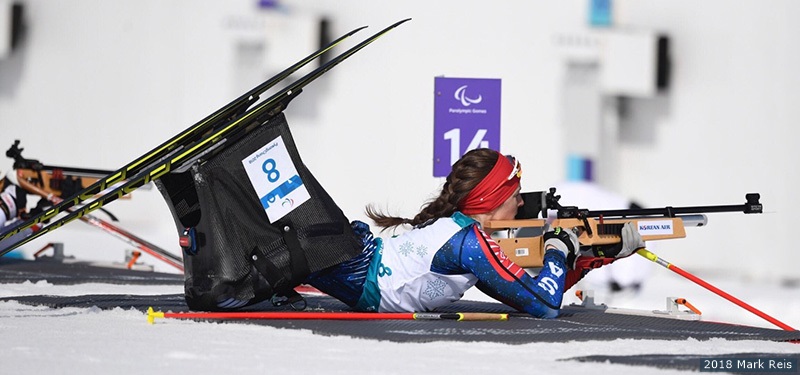A detailed photograph taken in winter 2018 by Mark Reese shows a woman participating in a shooting competition, possibly linked to the Special Olympics. The scene is set outdoors on a snowy field, indicated by the abundant snow and the woman's winter attire, including gloves. She is lying prone on a dark gray tarp or rug, with her legs partially obscured by a black mesh bag marked with the number 8. Above her head, a purple sign with the number 14 stands out against the white and blue buildings in the background. The woman is wearing a white shirt with royal blue sleeves and a red patch on her shoulder, suggesting some affiliation. Her brown hair is tied back in a braid, secured by a red fabric band and topped with glasses. She is holding a tan sniper rifle with a very long scope, supported by a metal pole on the right. The entire image is imbued with rich colors including purple, white, blue, red, black, and yellow, contributing to its vividness and detail.